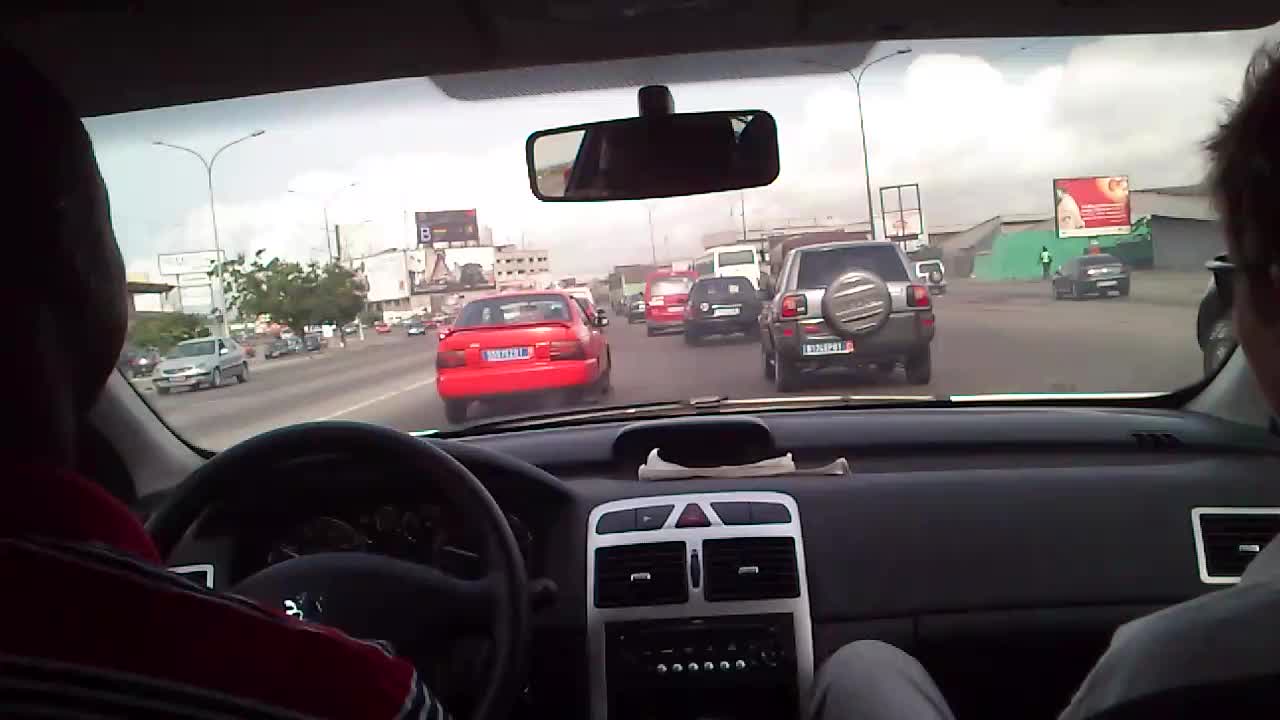The photograph is taken from the center back seat of a moving vehicle, providing a detailed view of the busy roadway ahead. The car's interior features two visible occupants: the driver in a red and black striped collared shirt and the passenger in a white shirt, viewed from behind. The dashboard is predominantly black with silver accents around the radio and ventilation systems, and includes two analog speedometers. The black steering wheel features a silver symbol in the center, and the control panel has numerous knobs.

The exterior view through the windshield shows a light and dark gray road teeming with traffic. Directly ahead, a red car is on the left and a gray SUV on the right, with several other cars in the distance and one car in the oncoming lane. On the left side of the road are buildings adorned with white and gray facades, some displaying large billboards. Dark green trees are also visible on this side. The right side showcases a mix of buildings, including a green one, and a red and white billboard sign, as well as a dark green tarp towards which an individual is walking. The sky above is overcast with storm clouds, adding a dreary atmosphere to the scene. The overall impression is one of a typical, bustling urban commute, with the car moving slowly through the dense traffic.